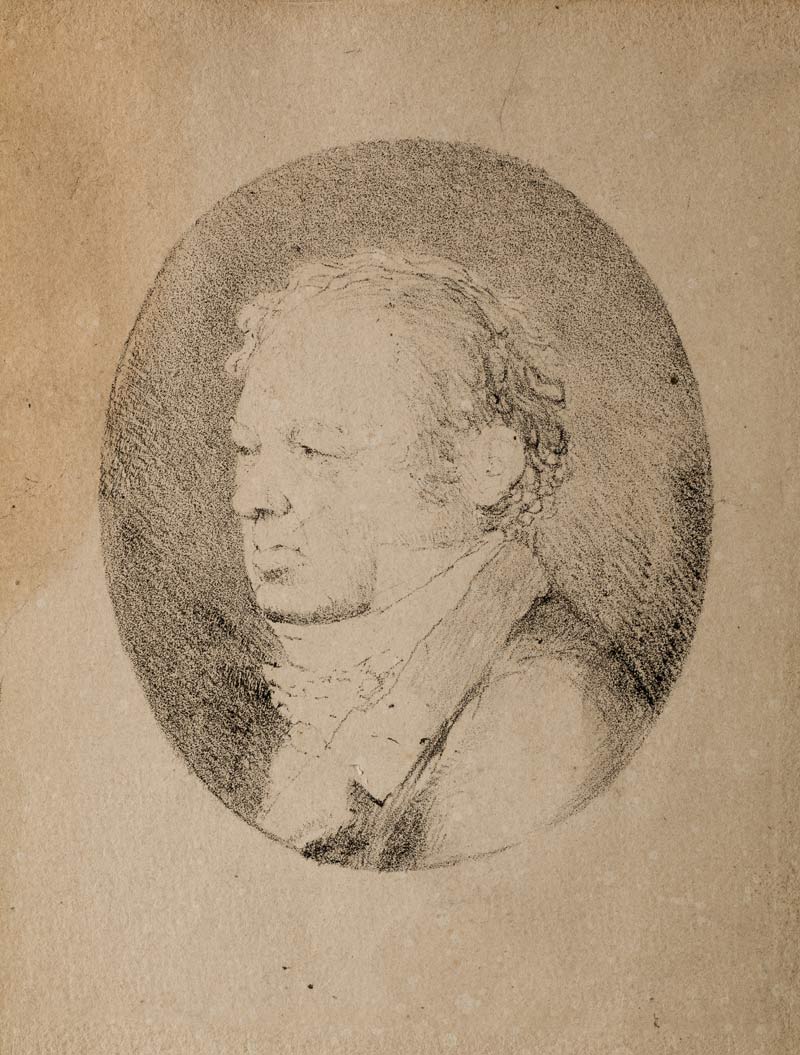This is a vertical rectangular image, depicting a detailed pencil sketch or charcoal drawing of a white man from the early 1800s. The drawing is positioned on an aged, light brown piece of paper that appears dirty and spotted, possibly due to the passage of time. In the center of the paper, a vertical oval frame encloses the portrait, reminiscent of the face of a coin. The man, captured in a near-profile view, has curly, receding hair around his ears and is wearing a dark suit coat, high-collared shirt, and an ascot tied around his neck. His expression is stern or neutral, with a noticeable scowl and eyes that seem half-closed, looking off to his right. His attire and the sketch's style suggest the setting is from the early 19th century. The background within the oval is darker, providing contrast that highlights the detailed features of the man's face and clothing.